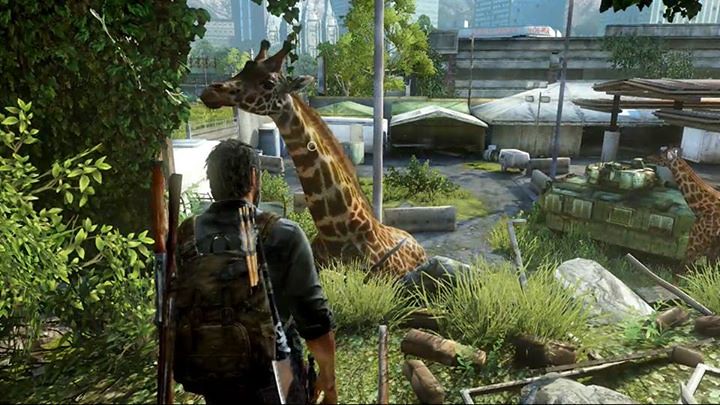This horizontal, rectangular, color image is a detailed screenshot from a video game, likely "The Last of Us." The scene shows a post-apocalyptic setting with an industrial park overtaken by nature. In the center, a large giraffe stands amidst scrub, brush, and scattered pieces of wood, with a smaller giraffe positioned to its lower right, further back in the frame. Deciduous trees occupy the left quarter of the image, adding to the overgrown environment. The background reveals a cityscape of dilapidated, burnt-out buildings, enhancing the sense of abandonment and decay. 

A man stands just left of center in dark gray clothing, including a rolled-up blue shirt, a scruffy beard, and short brown hair. He bears a camouflage backpack equipped with two rifles slung over his left shoulder, arrows, and an axe with its blade facing away on his right. The lack of visible facial details conveys a sense of mystery and survival. The scene captures the convergence of human survival and the reclaiming wilderness in a vividly detailed post-apocalyptic world.